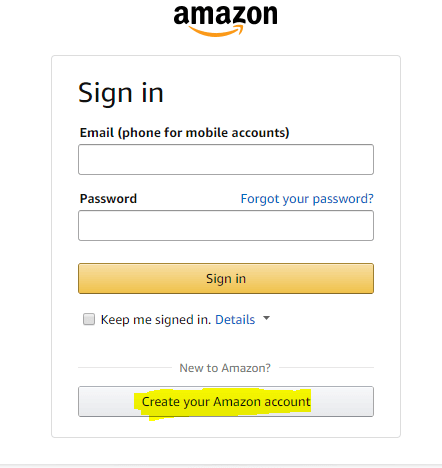The screenshot captures the Amazon sign-in page. At the top, prominently displayed is the Amazon logo, featuring lowercase black text and the signature orange smile that stretches from the 'A' to the 'Z'. 

The sign-in area is enclosed within a single-pixel gray border with subtly curved corners. Below the border, a slightly wider thin gray line accents the bottom space. At the top of the sign-in field, there's the text "Sign-In" in large black font.

Following this, in bold text, the word "Email" is presented, along with "phone for mobile accounts" in brackets. An input field for email or phone number is positioned below this label and is currently empty. 

Next, the word "Password" is shown, followed by another blank rectangular input field. Positioned to the right above this field is the blue hyperlink "Forgot your password."

An orange button featuring "Sign-In" in black text occupies the middle of this section, bordered by a gray outline. Beneath this button, aligned to the left, is an unchecked checkbox with the label "Keep me signed in" next to it, accompanied by the blue link text "Details" with a dropdown menu.

Dividing the section, a horizontal line spans the width, interrupted in the center by the phrase "New to Amazon?" enclosed within the two lines. 

Finally, at the bottom, another option asks, "Create your Amazon account." This text appears within a white field bordered by a gray outline, with a slight highlight effect over the content resembling a marker.

Overall, the composition is clean and functional, providing clear options for account sign-in and creation.